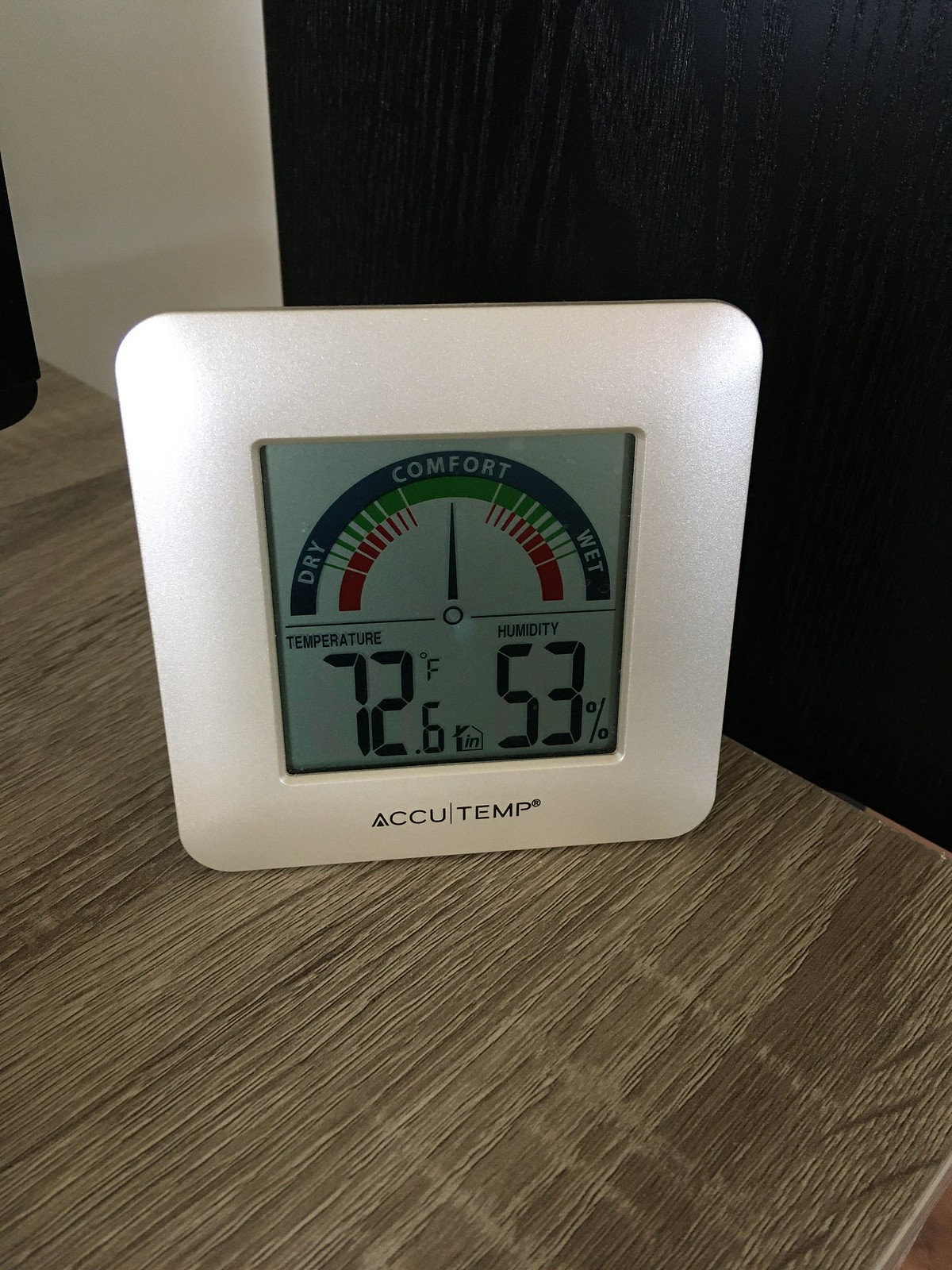A vertically-oriented photograph, likely taken with a smartphone or a budget camera, captures a dark brown wooden table in the foreground. On the table sits a digital temperature and humidity gauge, which is silver and white in color. The gauge displays a temperature of 72 degrees Fahrenheit and a humidity level of 53%. Additionally, it features indicators for "Dry," "Comfort," and "Wet" zones, accompanied by a small rotating arrow that points to the current conditions. The background consists of a plain white wall, and to the right of the gauge, there is a small black object whose details are unclear.